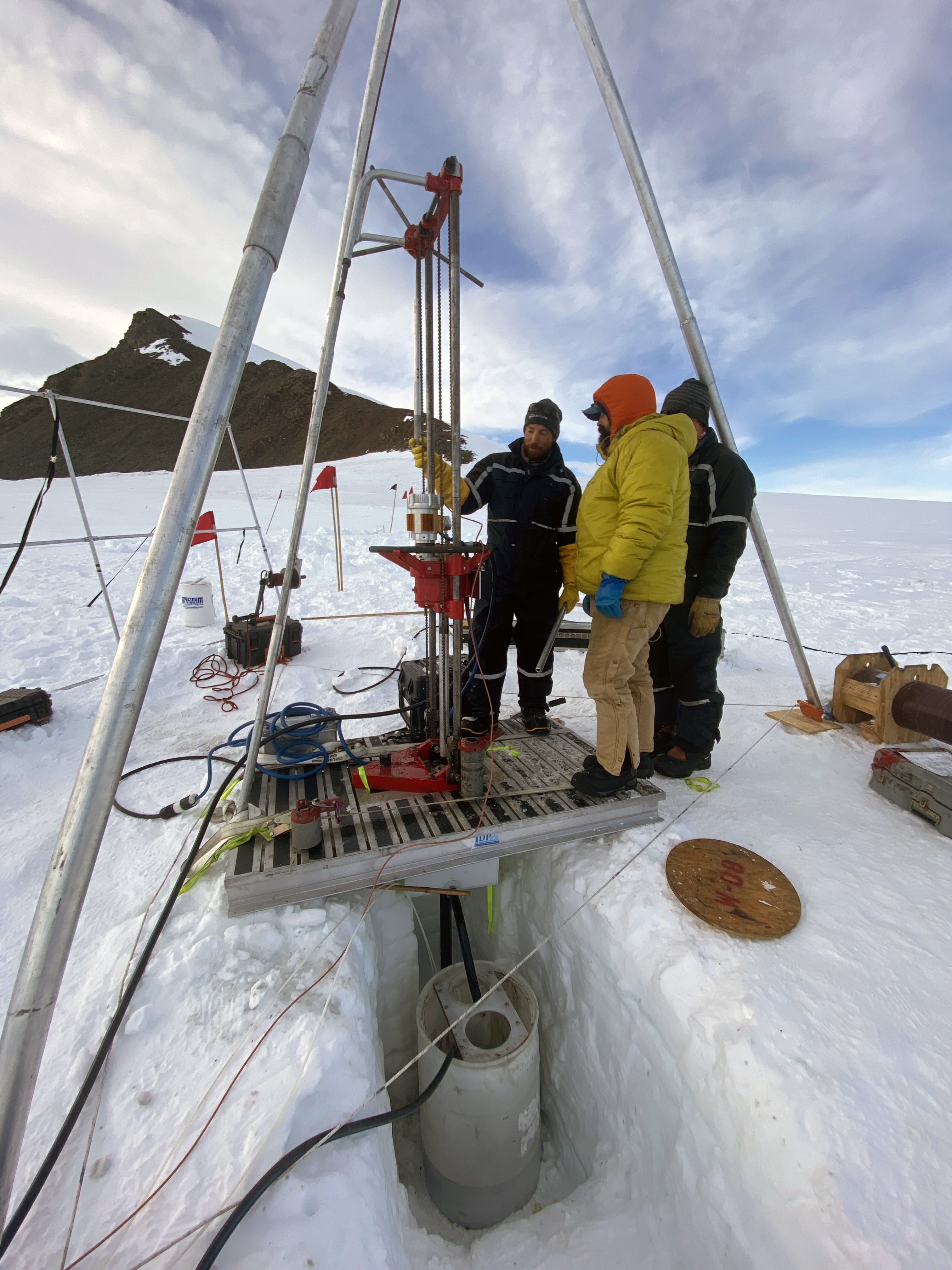In this captivating photo, three heavily bundled researchers are conducting an operation in a polar region, likely the Arctic or Antarctica, amid extremely cold conditions. They stand atop a metal platform erected on a landscape dominated by very deep, compacted snow. Each person is outfitted in thick jackets, full-body suits, hats, gloves, and heavy work boots to combat the frigid environment. The men focus intently on a piece of drilling equipment that extends approximately 15 feet into a meticulously carved-out section of the snow. A complex arrangement of metal tubing and hoses surrounds them, with one man gesturing towards the apparatus while the others observe attentively. Below the platform, a plastic tub is positioned, connected to the tubing, suggesting a potential research or drilling activity. In the backdrop, a rugged mountain with sparse snow patches rises against a cloudy yet partially blue sky, contributing to the harsh and remote setting of the scene.